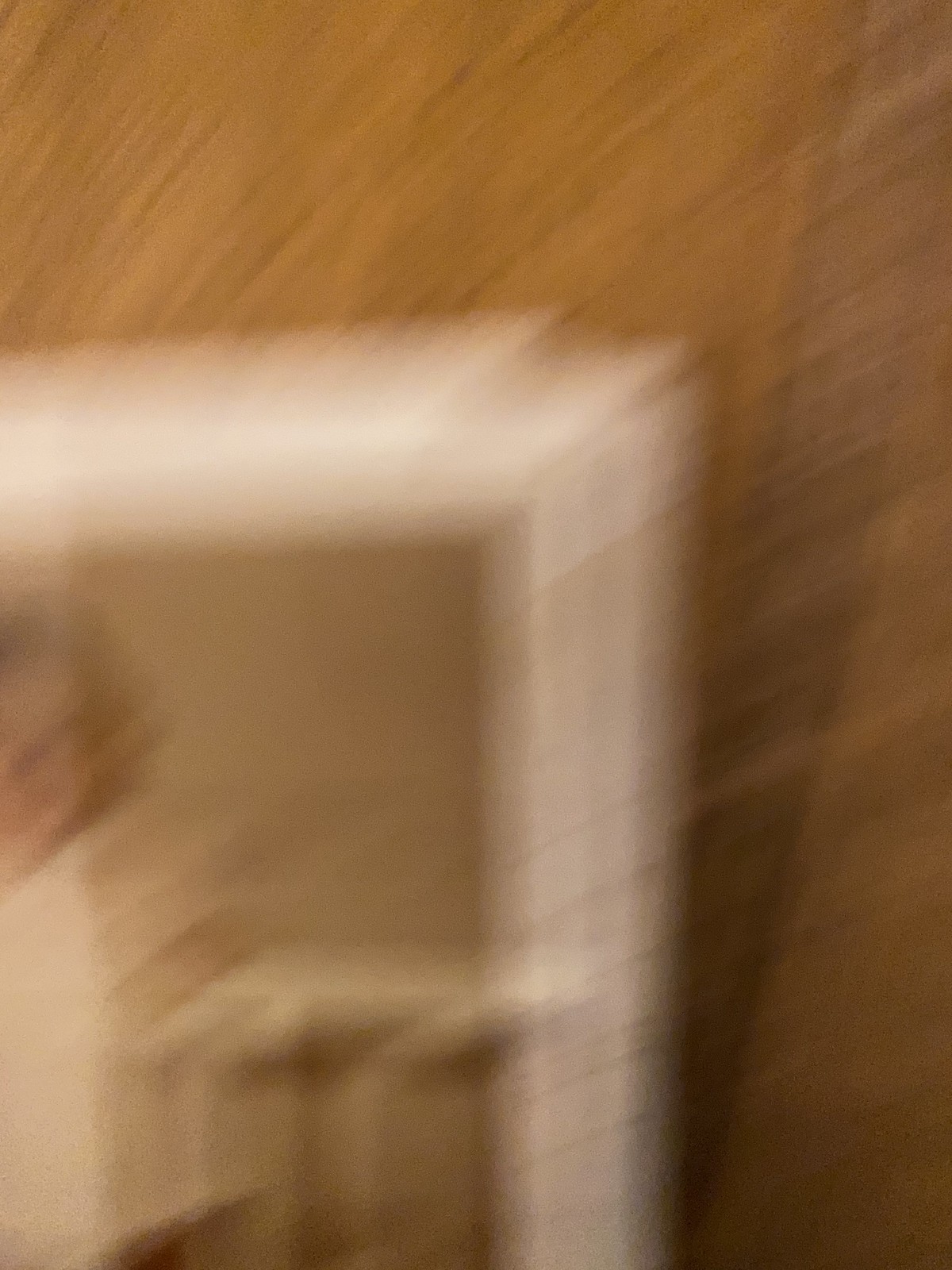This is a vertical, portrait-mode photograph characterized by significant motion blur, making it difficult to clearly identify its subjects. Central to the image appears to be a white picture frame or possibly a crib, with tan and white interiors accented by splotches of brown. The overall color palette of the photograph seems to include various shades of brown, ranging from dark chocolate brown to orangish-brown, particularly noticeable on the right side of the image. There are wisps and blurriness throughout, suggesting the camera was moved too quickly or the photographer tripped during the capture. This motion has obscured finer details, giving the entire scene an unfocused appearance. In the background, what seems to be wood paneling or a wooden table can be vaguely discerned, adding to the overall rustic yet unclear setting.